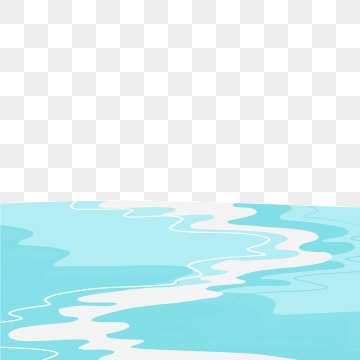The image features a top section adorned with a checkered pattern of white and pale blue squares, arranged in almost seven rows of eleven squares each. Below this patterned section is a detailed drawing of a river. The river illustration includes wave-like patterns in varying shades of blue, from dark blue to blue-green. A notable feature in the middle of the river is a stream of white water that flows vertically from top to bottom, creating a striking contrast against the surrounding wavy lines. The checkered pattern transitions into the river scene with an uneven cut, giving the image a dynamic composition. Overall, the image artfully combines geometric order and organic fluidity without any text, maintaining a focus on visual elements.